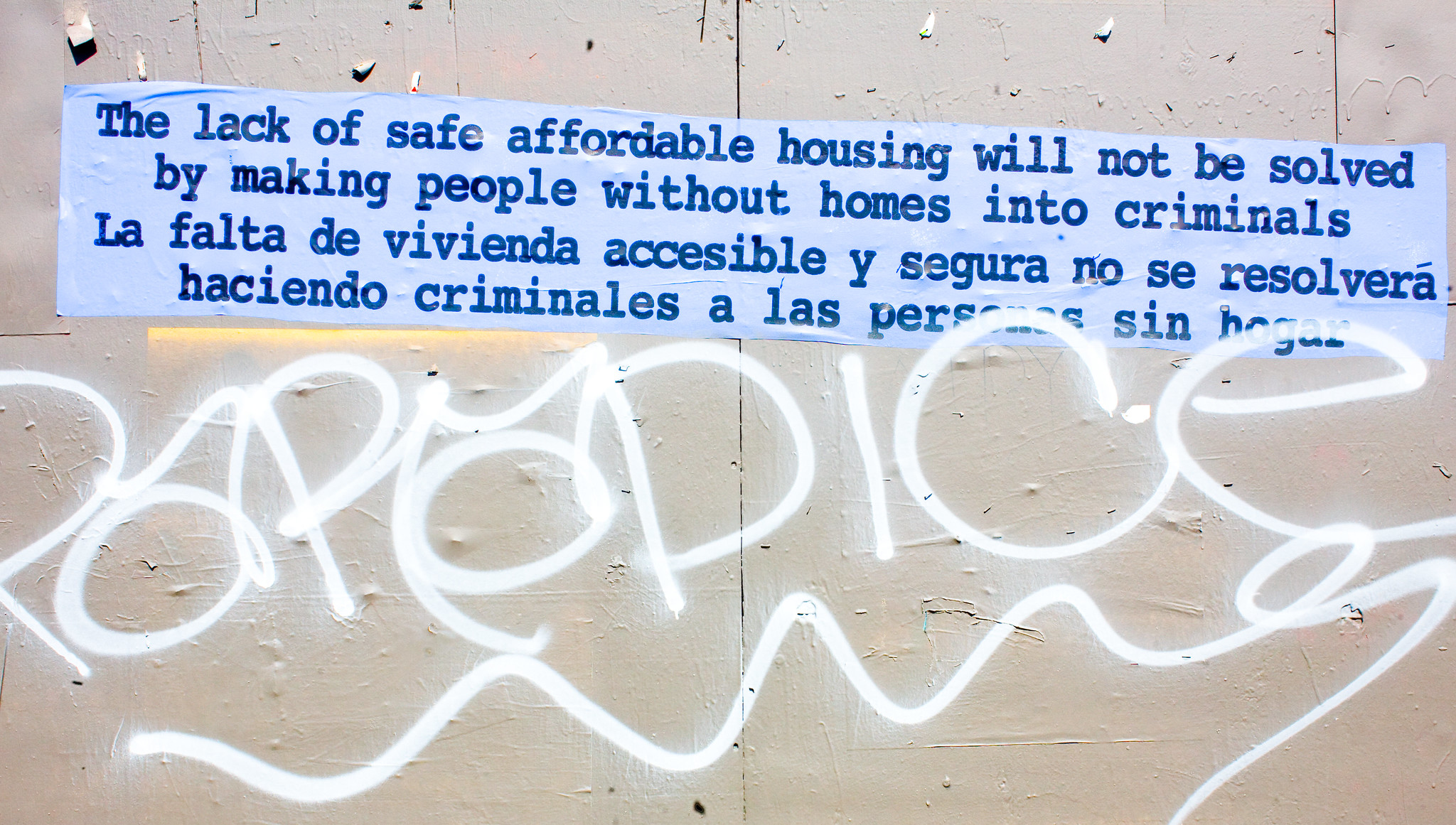The photograph captures an outdoor wall composed of irregular beige panels with flaking paint, adding a textured backdrop. At the bottom of the wall is white graffiti, potentially spelling "P-O-P-D-I-C-E," underlined with a squiggly line. Above the graffiti, a light blue rectangular sticker features a message in a typewriter font. The message reads: "The lack of safe affordable housing will not be solved by making people without homes into criminals." This is immediately followed by the Spanish translation: "La falta de vivienda accesible y segura no se resolverá haciendo criminales a las personas sin hogar." The image has a wider-than-tall orientation, reminiscent of the dimensions of a high-definition television, and gives off a somewhat authoritarian and uninviting vibe, possibly akin to a government notice. The text and graphical elements vary in shades of blue, adding to the visual complexity of the scene.